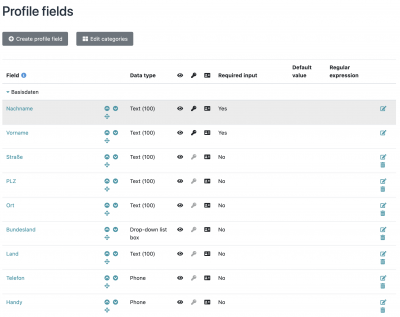The image depicts a small and slightly blurry user interface, likely of a profile creation tool. At the top left of the interface, the header "Profile Fields" is clearly visible. Below this header, there are two gray buttons: the left button is labeled "Create Profile Field," while the right one is labeled "Edit Categories."

The main part of the image features a tabular list of profile fields. Each row in the table represents a different field, with the following column headers:
1. Field Name (text is blue)
2. Data Type
3. - 
4. Required Input (Yes/No)
5. Default Value
6. Regular Expression
7. - 
8. - 
9. Edit (represented by a pen and paper icon on the far right of each row, indicating that clicking it allows editing of that particular field)

The table and text are set against a white background. Although the text's small size and blurriness make it hard to read the exact contents of the fields, the blue text likely corresponds to the different profile fields listed. The table’s organizational structure is demarcated with black text and borders for easy readability.